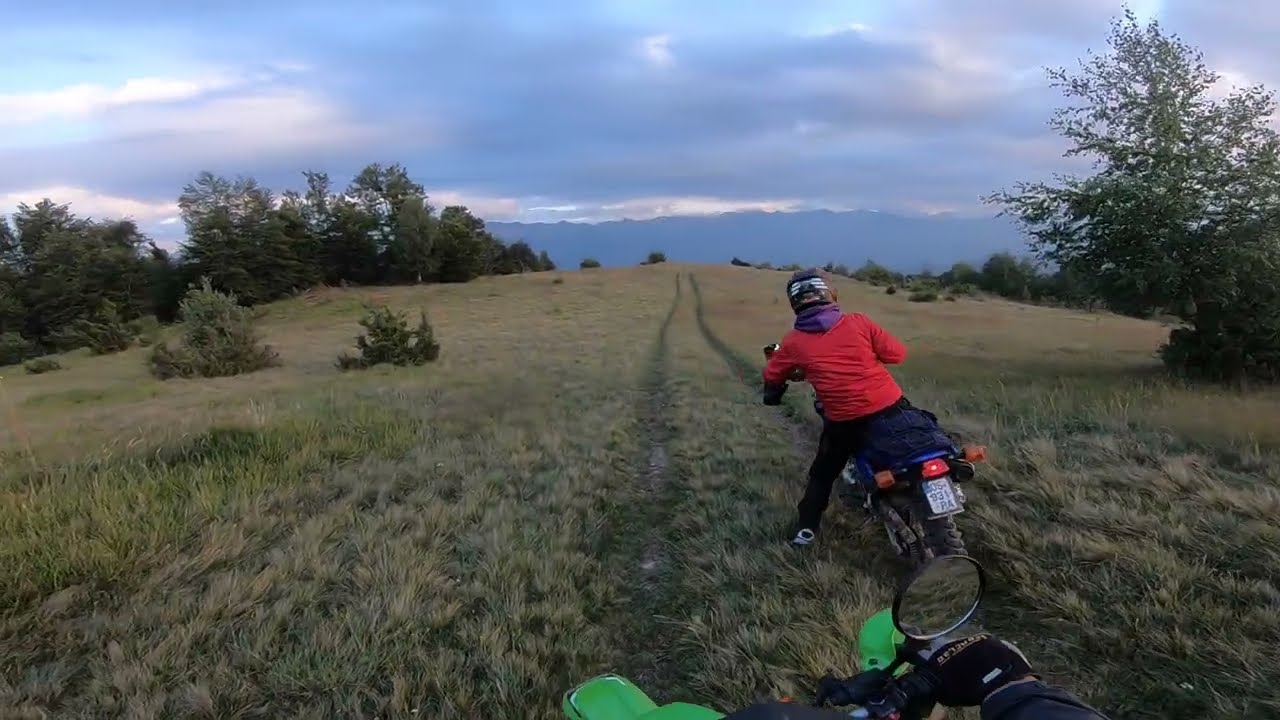The photograph captures a dynamic scene of two individuals riding dirt bikes through an expansive, grassy field. The image appears to be taken from a GoPro mounted on one of the riders' helmets, providing a point-of-view shot that includes a partial view of the handlebars and a gloved hand gripping the handlebar of a light white and lime green dirt bike. Ahead, another rider on a blue dirt bike, dressed in an orange-red jacket with a purple hood, black pants, and a black helmet, is following a set of double tire tracks that cut through the medium-length yellow grass. The narrow dirt path stretches from the bottom center of the frame into the horizon, flanked by scattered trees and low bushes. In the distance, hills or mountains are faintly visible under a mostly cloudy sky that takes up the upper half of the image, completing the sense of an adventure in the middle of untamed nature.